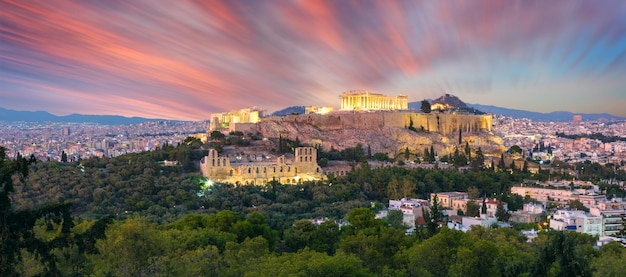In this breathtaking panorama, an aerial view captures the sun rising, casting a serene glow of pinks, purples, oranges, and grays across the sky, streaked with mesmerizing clouds. The scene is dominated by a verdant foreground of densely packed, leafy hardwood trees, suggesting the lushness of spring or summer. Just beyond the treetops, the city stretches out, a sprawling expanse of white and grey buildings. An imposing structure capped with yellowish columns stands regally on a brown cliff or plateau, evoking the grandeur of an ancient Greek temple, potentially the Art Museum in Philadelphia or the Acropolis. This ancient, columned edifice illuminates the scene, bestowing a timeless quality. The horizon showcases more city buildings bathed in the soft sun's light, completing a picturesque and tranquil tableau.